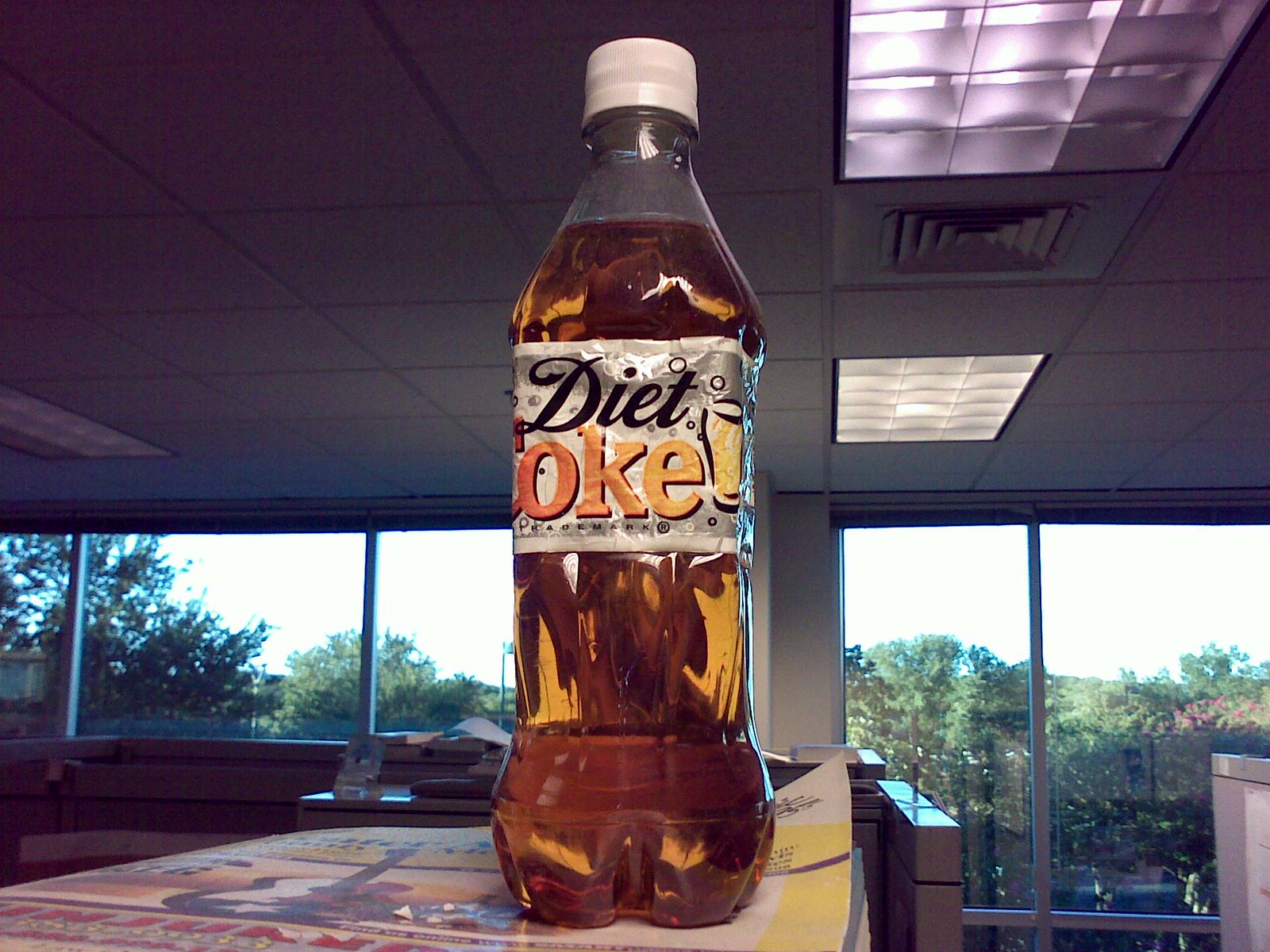This photograph captures a seemingly commercial office area, though it could potentially be an apartment. The space is characterized by its distinct decor, stairway construction, and acoustical ceiling tiles that give it a commercial vibe. The ceiling features recessed fluorescent lighting with diffusers and a ventilation grate. 

In the foreground, there is a table where an interesting arrangement draws attention. Resting on top of a softcover manual or book that also supports an acoustic guitar, there is a strikingly deformed plastic bottle of Diet Coke. The bottle, still sealed with its white cap, appears to have been crushed into a square shape, likely from being squashed at the bottom of a transport box or under a stack of heavy items. The label on the bottle shows clear signs of damage, indicating the bottle has endured significant pressure. This peculiar square bottle of Diet Coke sits prominently atop the manual, adding a curious focal point to the image.